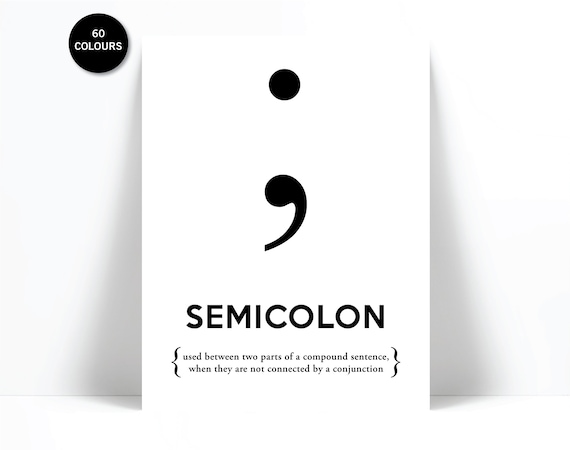The image depicts a white card leaning at an angle against a white wall, casting a triangular shadow on either side. The card features a prominent black semicolon symbol, followed by the word "SEMICOLON" in large capital letters. Directly below this, in smaller font and enclosed in brackets, is the explanatory text: "used between two parts of a compound sentence, when they are not connected by a conjunction." In the top left corner of the card, there is a black dot containing the text "60 colours," spelled in British English (C-O-L-O-U-R-S), written in white letters. The overall style is graphic and minimalistic, with clear delineation of elements and shadows that add depth to the simple yet informative design.